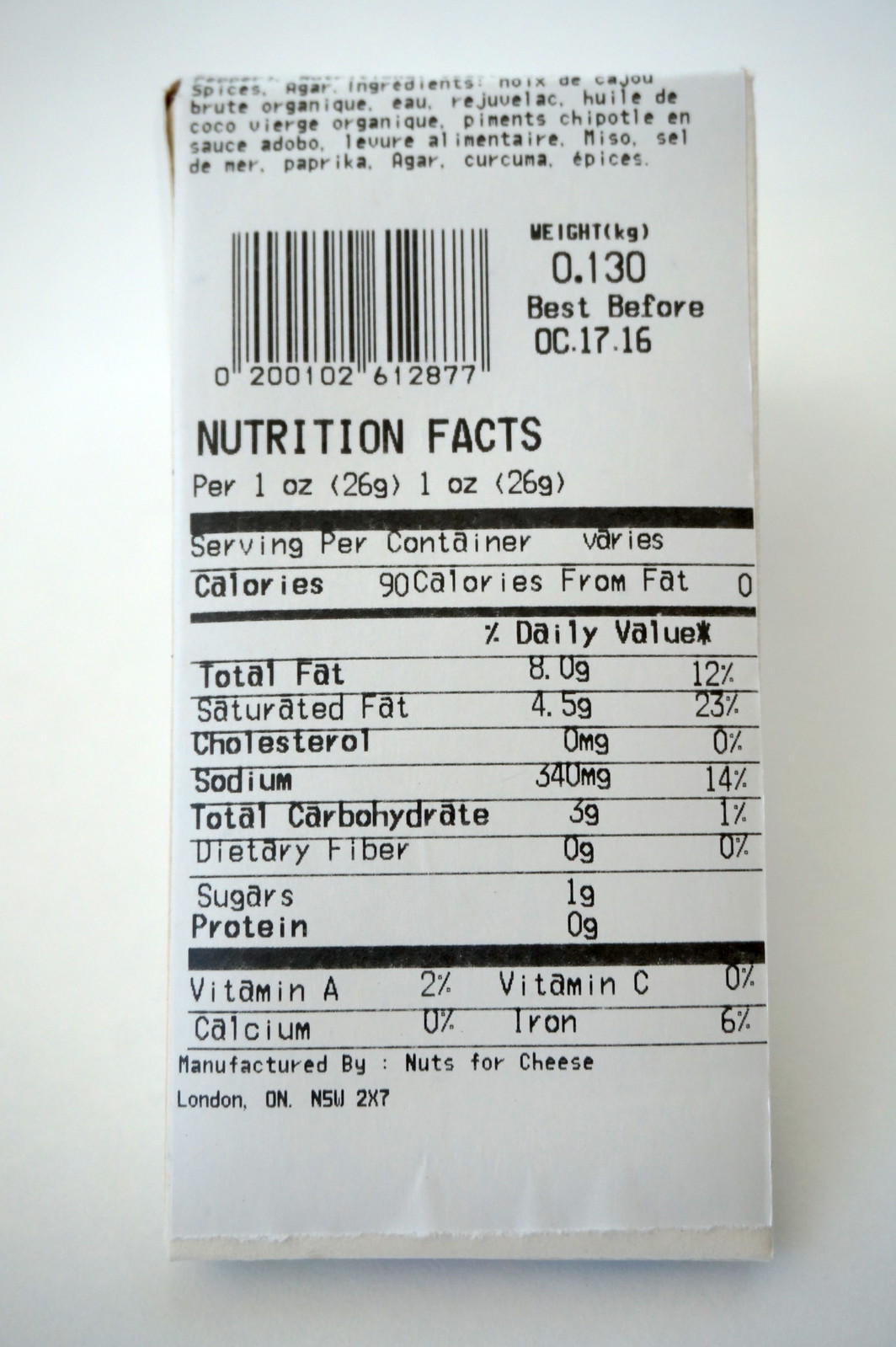On an all-white background, possibly resembling a calendar, a detailed nutrition facts label is displayed. At the top of the label, the list of ingredients is visible, although specifics cannot be determined from the image. Below the ingredient list is a barcode accompanied by its corresponding numerical code. The packaging details continue with the item’s weight provided in kilograms, followed by a "Best Before" date of October 17, 2016. 

The nutritional information indicates that a single serving size is one ounce, though the number of servings per container varies. The label specifies that one serving contains:

- 96 calories
- 0 grams of total fat
- 8 grams of saturated fat
- 4.5 grams of trans fat
- 0 mg of cholesterol
- 340 mg of sodium
- 3 grams of total carbohydrates
- 0 grams of dietary fiber
- 1 gram of sugars
- 0 grams of protein

Additionally, the label lists vitamin A, vitamin C, iron, and calcium, though exact quantities for these nutrients are not provided.